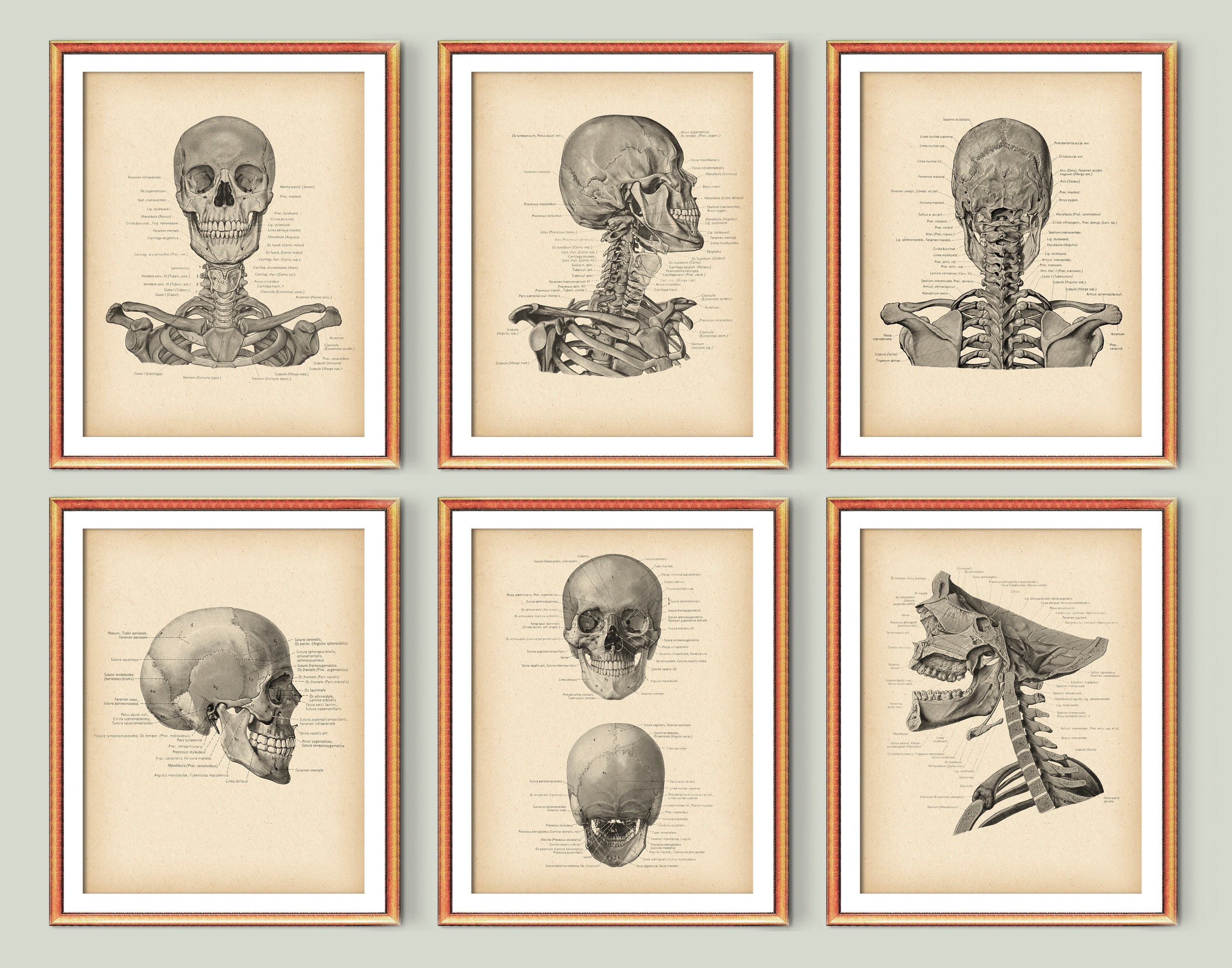This is a collection of six scientific drawings, framed and matted, each enclosed in a golden-orange wooden frame with white matte borders. The illustrations are monochromatic, rendered on a yellowish parchment-like paper, and depict various anatomical views of the human skull and shoulder areas. Each image is meticulously labeled with different body parts and bones, although the resolution prevents the labels from being easily readable. 

The top left frame contains a front view of the skull and shoulders. Below it, the second frame displays a side profile of the skull facing right. The middle frame on the top row illustrates the back view of the skull and shoulder blades. The bottom row begins on the left with another side profile of the skull. Next to it, the second frame shows a detailed front view of the skull. The final frame on the bottom right offers a cross-sectional view of the spine and skull. All six frames are arranged on a grayish wall, presenting a comprehensive visual study of the skull from multiple perspectives.